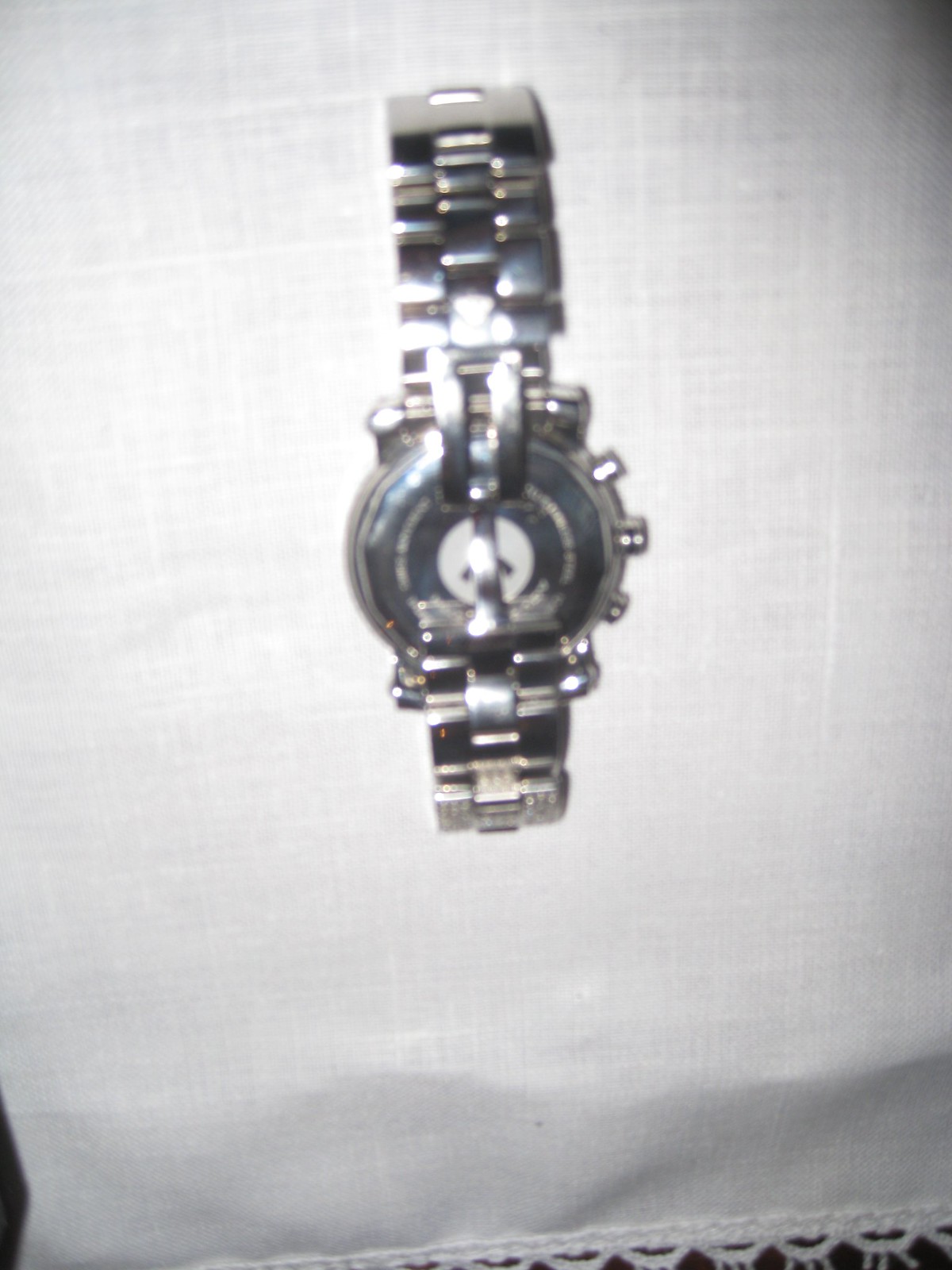This detailed photograph showcases a silver men's watch, which appears to be the back side, resting on a piece of white fabric with a fringe of small circular rings along the bottom edge. The cloth, which could be linen or another type of soft material, is slightly rumpled towards the bottom, giving it a textured appearance. The watch's band, made of wide silver links, is slightly open, with the metal clasp overlaying part of the watch's back. The back of the watch features a conspicuous white circle in the center, possibly housing some text or designs that are partially obscured by the band's position. Additionally, three small knobs, likely for winding or adjusting the watch, protrude from the right-hand side. The image is somewhat zoomed in with a light glare, providing a close-up view of the intricate details of the watch and the soft fabric it rests on.